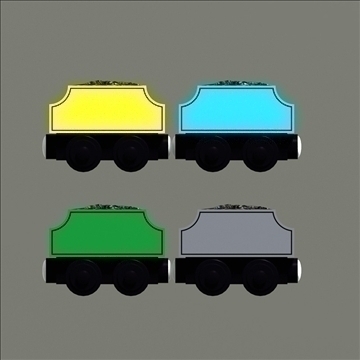The image is a computer-generated graphic featuring four identical objects that resemble train cars or wagons, arranged in a neat square formation. Each object sits on a black base with two circles resembling wheels, enhancing their cartoonish, vehicle-like appearance. The train cars consist of rectangles with cut top corners, giving them a slightly hexagonal shape. Positioned perfectly in the center of a plain, slate grey background, the train cars are presented in two rows of two. From top left to bottom right, the colors of the train cars are yellow, light blue, green, and greyish-black, and they appear to be loaded with a texture that might represent iron ore or rocks spilling out from the top. The overall quality and simplicity of the graphics suggest that the image might have been created by a child.